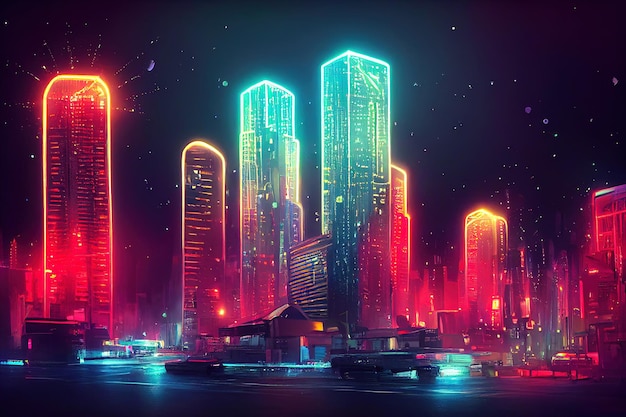This fantasy-style drawing depicts a neon-lit cityscape at night, evocative of a retro-futuristic downtown, reminiscent of 80s video game or movie cover art. The sky is a deep blue-black, dotted with white stars that glow faintly. Dominating the scene are several large buildings and towering skyscrapers, bathed in electric neon hues. The central structures are illuminated in vibrant blue outlined with light blue, while others are highlighted in striking dark pink or orange, with bright orange outlines. These vivid colors create a garish yet captivating contrast against the dark night sky.

Below the glowing towers, the foreground features a dark, seemingly wet street that reflects the neon light above, mimicking a rain-soaked surface. Blurry figures, possibly futuristic vehicles, add a dynamic element to the scene. A couple of low-rise buildings nestled in front of the skyscrapers hint at a varied architectural landscape. Small structures, possibly homes, and blurred elements suggest boats with subtle blue lighting blend into the composition. This detailed rendering, strikingly detailed and complex, brings forth a nostalgic nod to neon aesthetics and a futuristic vision.